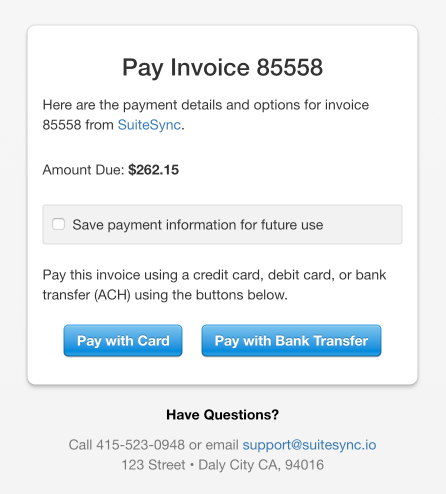**Detailed Caption:**

The image features a light gray rectangular background with a white square near the top. Within this white square, the text "Pay Invoice 85558" is prominently displayed. Below that, it states, "Here are the payment details and options for invoice 85558 from Sweet Sink." The company name "Sweet Sink" is highlighted in blue. Following a period in black, the text "Amount Due: $262.15" is shown.

Further down, within another light gray rectangle, there is a small white square containing the option "Save payment information for future use." Below this, the image instructs, "Pay this invoice using a credit card, debit card, or bank transfer (ACH) using the buttons below."

Two blue rectangles are positioned beneath this text, the first labeled "Pay with Card" and the second, longer rectangle labeled "Pay with Bank Transfer." 

At the bottom of the image, the contact information is provided: "Have questions? Call 415-523-0948 or email support@sweetsink.io." The address "123 Street, Daly City, CA, 94016" is listed at the end.